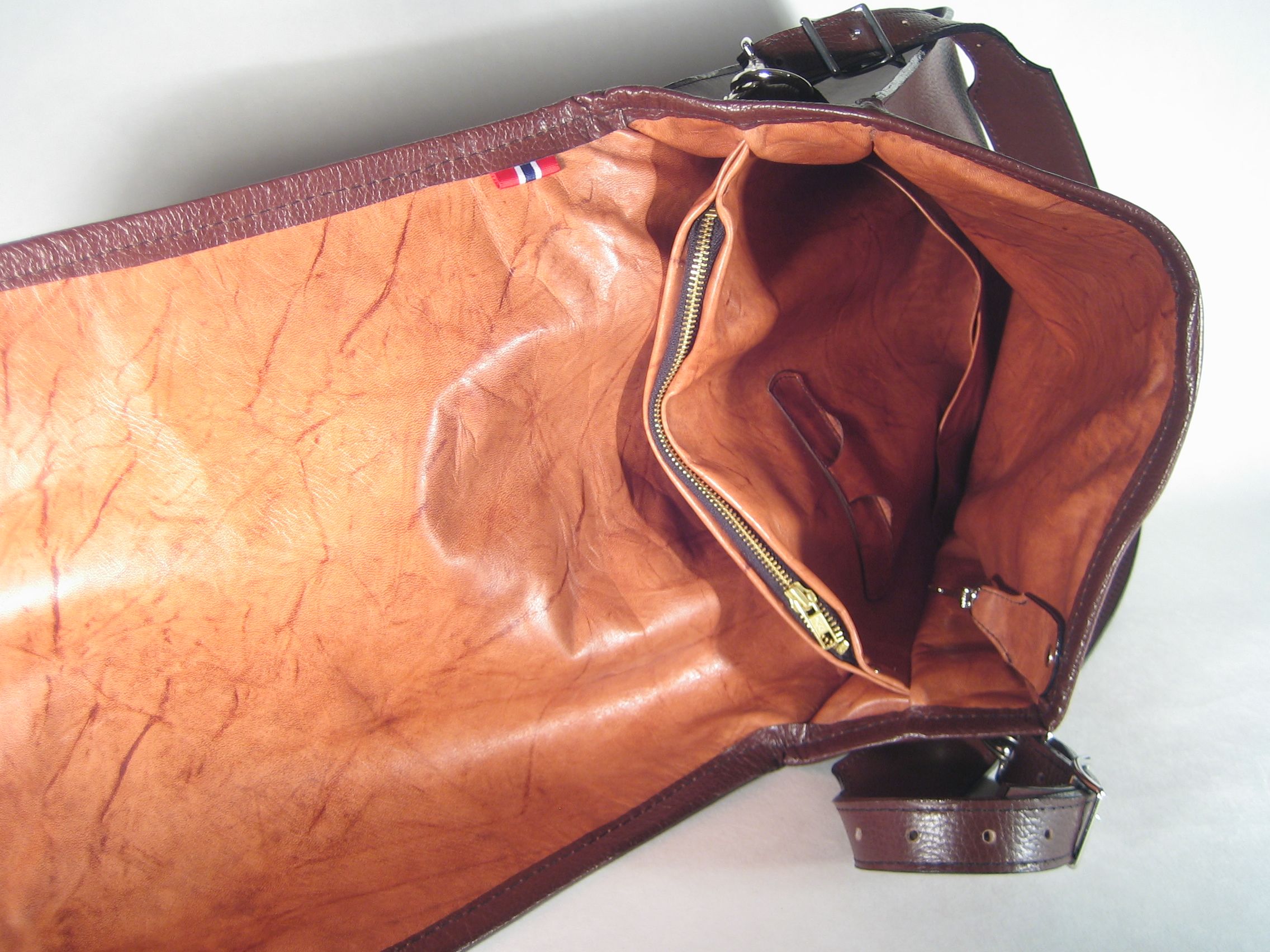The image displays a tan-brown handbag or satchel positioned diagonally from the bottom left to the upper right on a white background, casting a noticeable shadow. The bag, made of PU synthetic leather, has an open flap extending toward the left corner and edge of the image. Its interior features a zipped compartment on the left and another divider or pocket on the right. The handbag strap is adjustable brown leather with punched holes for the buckle. The bag's colors include tan, brown, gold, red, white, blue, and a hint of silver, suggesting the photo captures a casual, amateur styling, likely shared for social media.